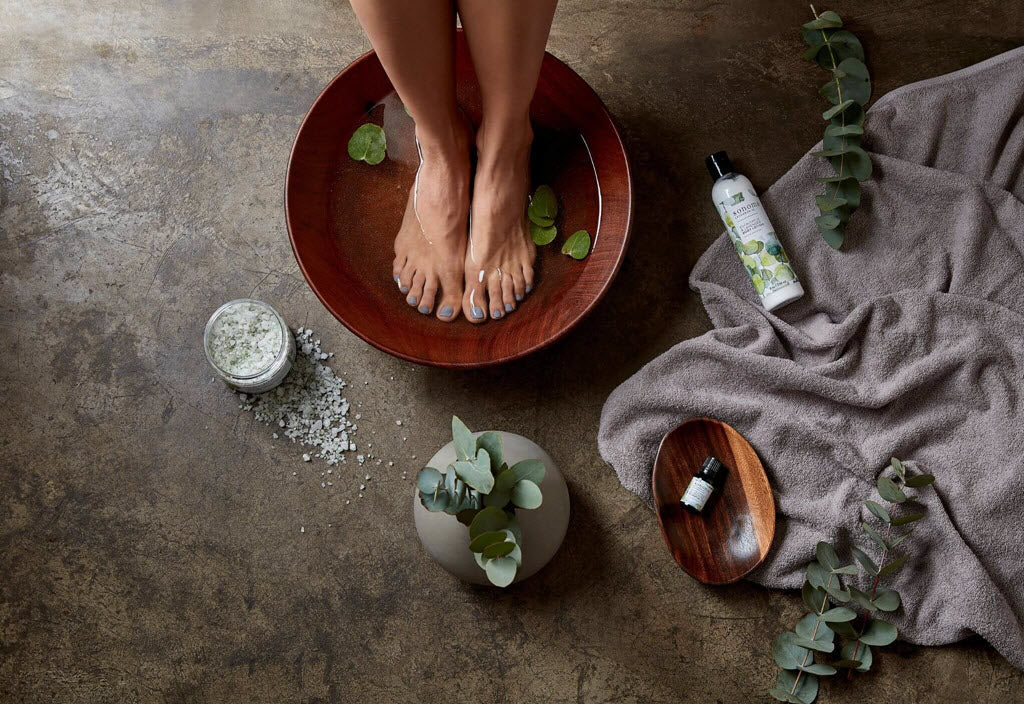The image is a detailed photograph depicting a serene home spa setup. Central to the scene is a large wooden bowl—possibly teak or cherry wood—filled with water, in which a person, presumably a white woman, is soaking her feet. Her toenails are painted in a light bluish-purplish pastel shade. Green leaves, possibly eucalyptus, float in the water. Surrounding the bowl is a well-arranged collection of spa items: to the right, a gray or purplish towel on which rests a white bottle with a black cap, likely containing body lotion by the brand Sonoma. Adjacent to it lies another small bottle, potentially shampoo or soap, and a leafy branch extending out of the frame. Additionally, a small, dark-colored glass bottle with a label sits in a wooden bowl on the towel. To the left of the large bowl, there's a squat, light-colored vase housing another leafy plant, and next to it, a jar of coarse sea or Epsom salt, some of which has spilled onto the dark, possibly stone or marble floor. The scene is completed with scattered sprigs of green leaves, creating a calming and organic ambiance.